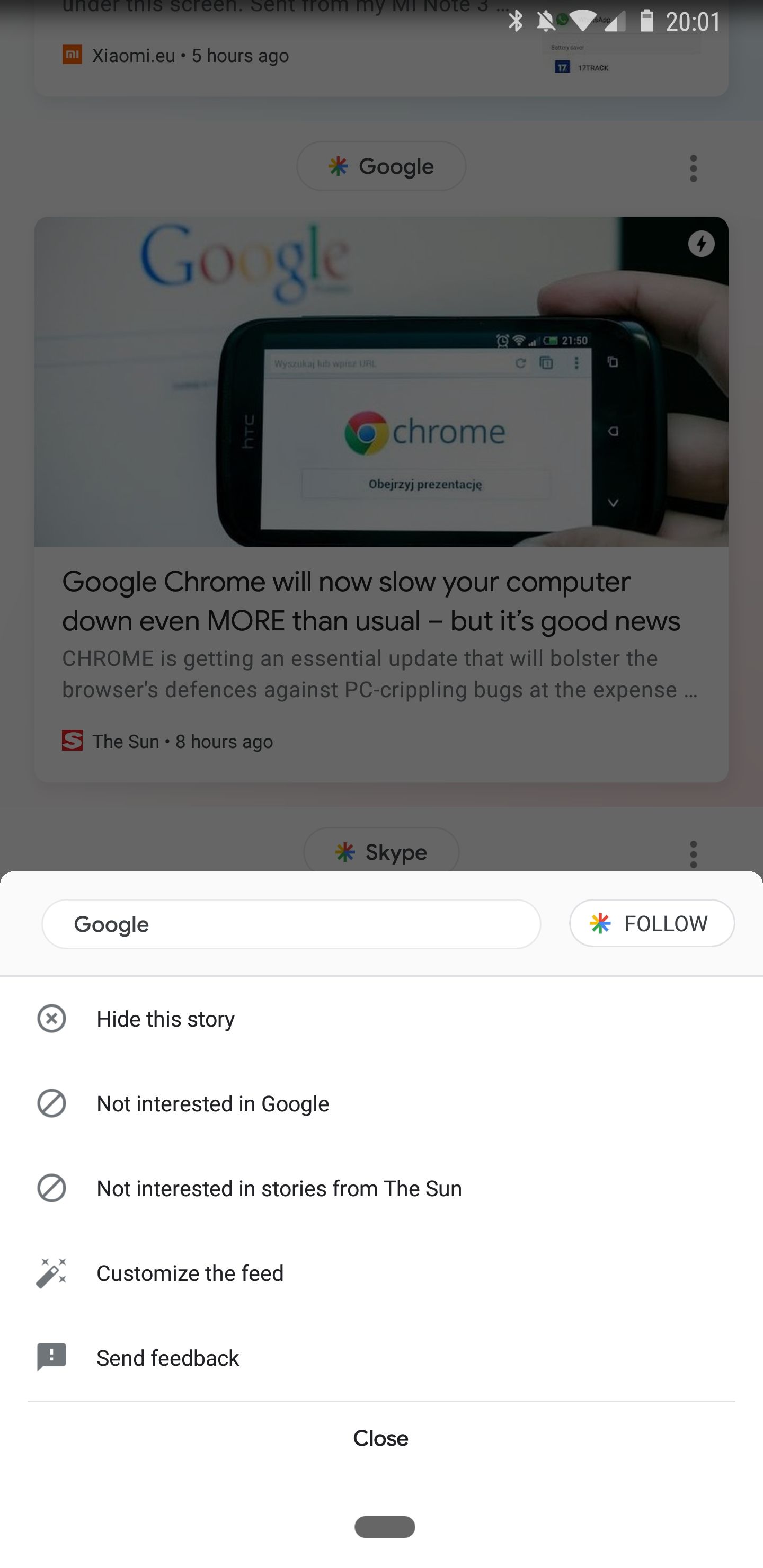Screenshot of a Xiaomi.EU Smartphone Interface

This image is a screenshot from a Xiaomi smartphone displaying a Google search page with an overlay of the phone’s notification center. The screenshot exhibits a faint grayish tint across the screen, possibly indicating the presence of an active notification or system feature.

At the top of the screen, the status bar includes various icons: Bluetooth, notification, Wi-Fi, and battery indicators, alongside a timestamp reading "20:01." Above the main content, a text element reads "xiaomi.eu - 5 hours ago."

The central portion of the screen features Google's homepage with its recognizable logo positioned on the left and a trio of vertical dots on the right, representing more options. Below this, there's an embedded image depicting Google's homepage on both a computer monitor and a smartphone. Superimposed on this image is a line of text written in a foreign language, difficult to interpret, regarding Google Chrome.

Further down, an informational banner states: “Google Chrome will now slow your computer down even more. Chrome is getting an essential update that will bolster the browser’s defenses against PC-crippling bugs at the expense...” This text is anchored by The Sun’s logo, which mentions the article was published 8 hours ago.

Beneath the article preview, there is a search bar within which the word "Google" is typed. Below this search bar is a button labeled "Follow," adjacent to which is an 'X' icon for dismissing the story. Options labeled "Hide this story" and "Not interested in stories from The Sun" follow, paired with respective symbols indicating these actions. Additional interactive elements, including buttons for customizing the feed, a warning icon, chat functions, and options for sending feedback, are also visible.

The bottom of the screenshot shows the typical navigation buttons, including a "Close" button and a home icon, signaling the end of the interface display.